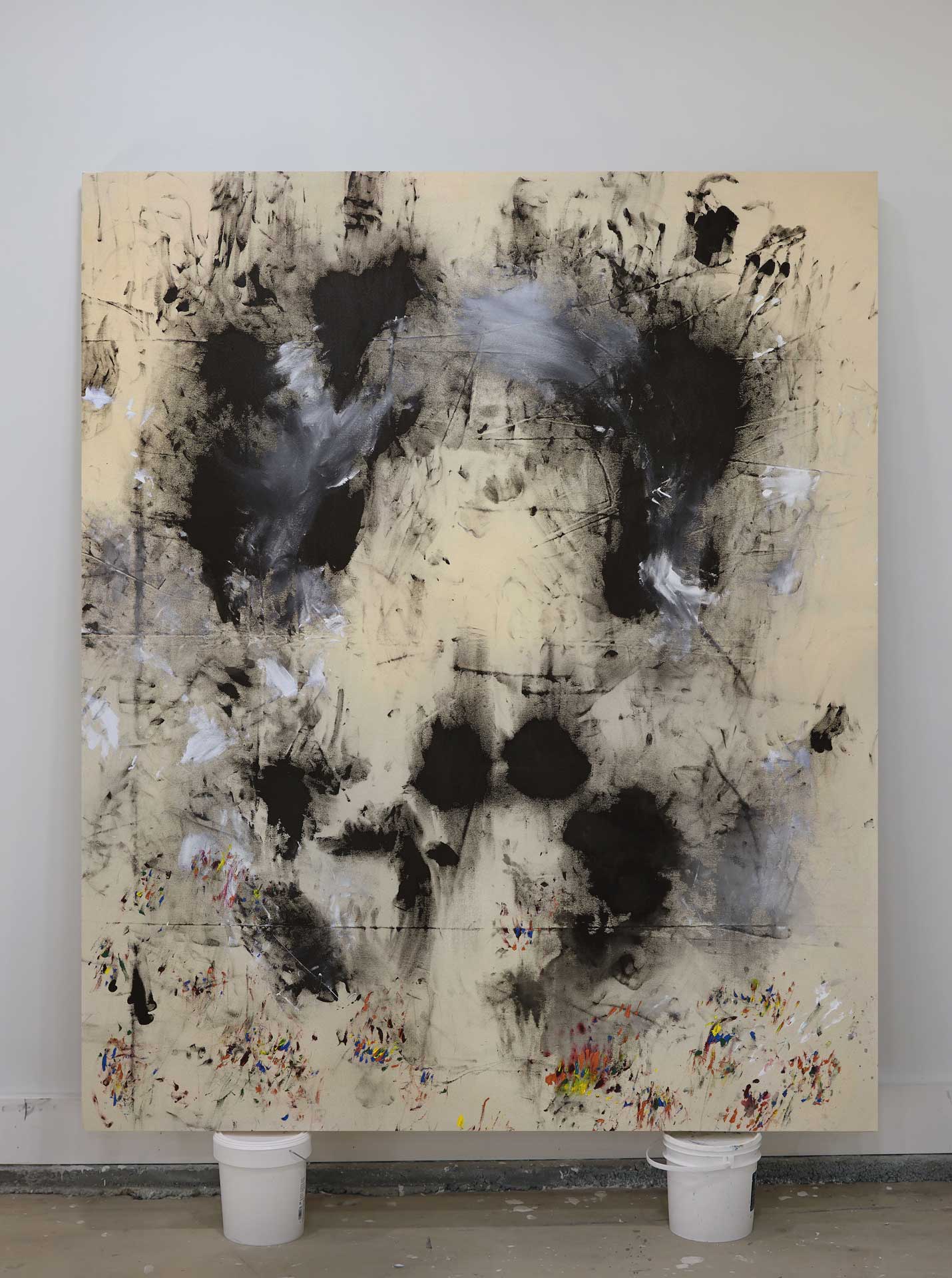In the image, a large canvas, resembling a painter's drop cloth, is propped up against a plain white wall. It rests on two white plastic buckets that are set on the floor, which appears to be a nondescript, off-white or grayish shade. The canvas is predominantly a light tan color and features an array of paint splotches and smudges. At the top of the canvas, there are substantial black blotches intermixed with smaller white spots. As the eye moves downward, these black and white smudges become less dense, giving way to a diverse array of colors near the bottom. Small, vivid splashes of yellow, red, blue, and orange scatter across the lower section, resembling a rainbow of colorful dots and strokes, in stark contrast to the monochromatic upper half. The painting exudes an abstract, expressionist feel, with its random yet intentional distribution of colors and forms.